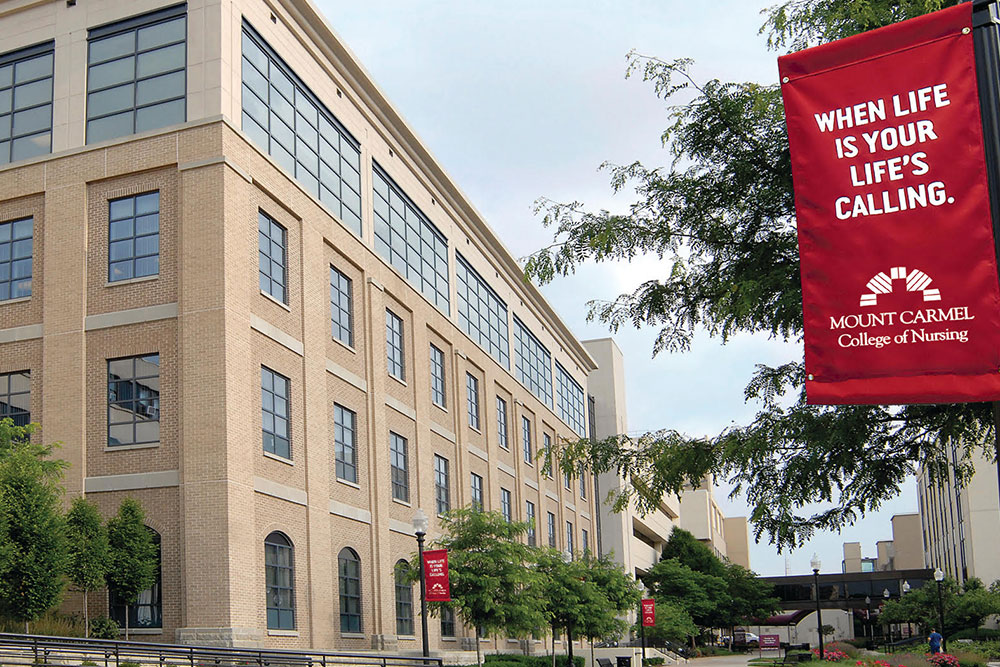The horizontally aligned rectangular photograph, taken outside during the daytime under blue skies, captures a bustling street view of a college campus, likely Mount Carmel College of Nursing, as indicated by the repeating red banners. These banners, with white text reading "When Life is Your Life's Calling" and "Mount Carmel College of Nursing," are prominently displayed on black poles along the sidewalk.

On the left side of the image, there is a large, four-story, tan-colored brick building that appears to be recently constructed. This structure features arched windows on the ground floor, vertical rectangular windows on the middle floors, and large horizontal rectangular sections of windows at the top. A series of smaller trees are planted in front of it, adding a touch of greenery to the scene.

Across the street on the right side, similar light-beige brick buildings continue, suggesting that they are part of the same campus. The right side also features a flower-lined walkway that extends into the distance, further enhancing the collegiate atmosphere. Also visible in the lower left corner is a black railing that runs across the sidewalk area, contributing to the well-organized and inviting environment of this academic setting.